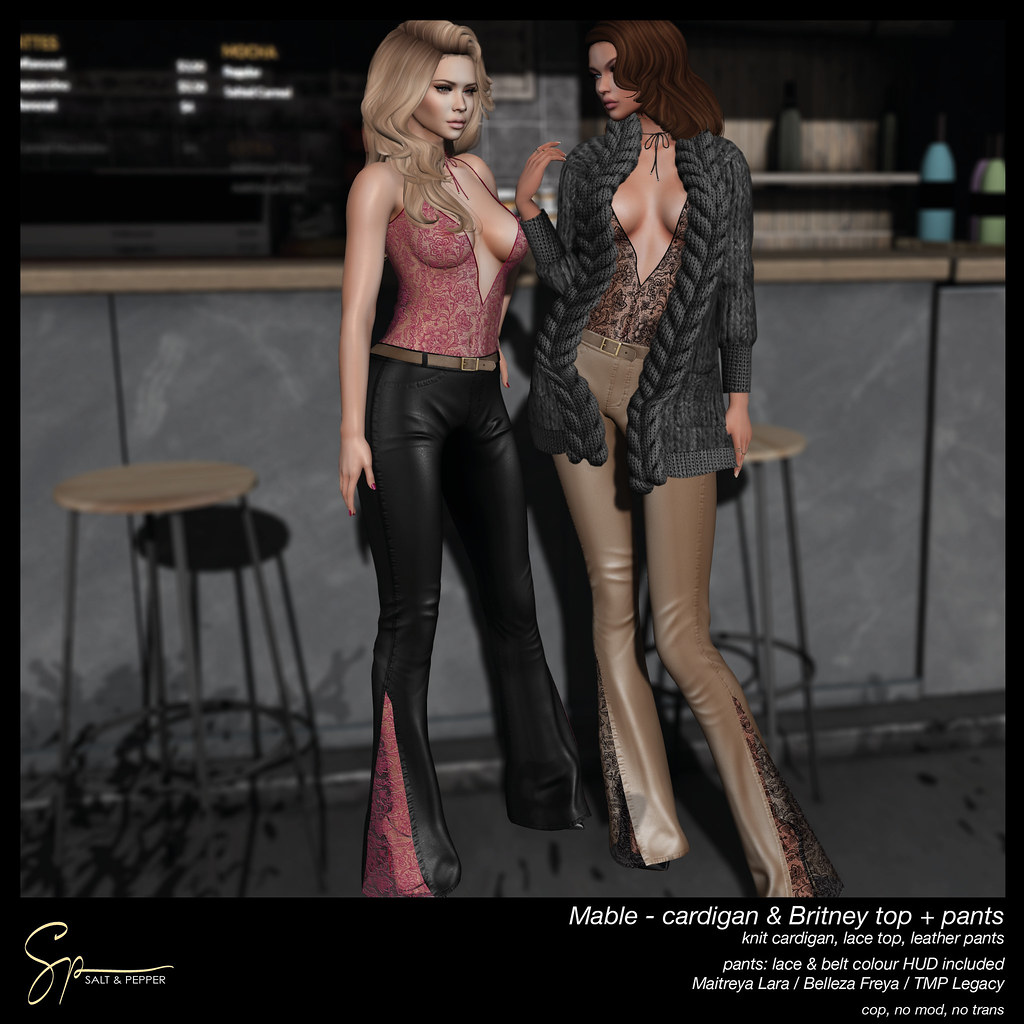The image depicts a detailed, computer-generated, in-game screenshot akin to The Sims, showcasing two cartoon-like 3D-rendered women in a bar setting with two bar stools in the background. On the left is a blonde, white woman wearing a revealing red lace top that showcases her cleavage, paired with tight black leather pants. On the right is a slightly darker-skinned woman with brown hair, wearing a long black knit cardigan over her lace top, complemented by brown pants. Both outfits highlight detailed fashion elements with mentions of Mabel Cardigan and Brittany Top plus Pants, reflecting sophisticated textures like lace and leather. The bottom right of the image features descriptive white text detailing the clothing items: knit cardigan, lace top, and leather pants, with additional information about included HUDs for customizing lace and belt colors. The text also lists compatible body shapes: Maitreya, Laura, Beleza, Freya, TMP, and Legacy, as well as item attributes, including Copy, No Modify, and No Transfer permissions. At the bottom left of the image, there's a watermark in yellow font reading "salt and pepper."